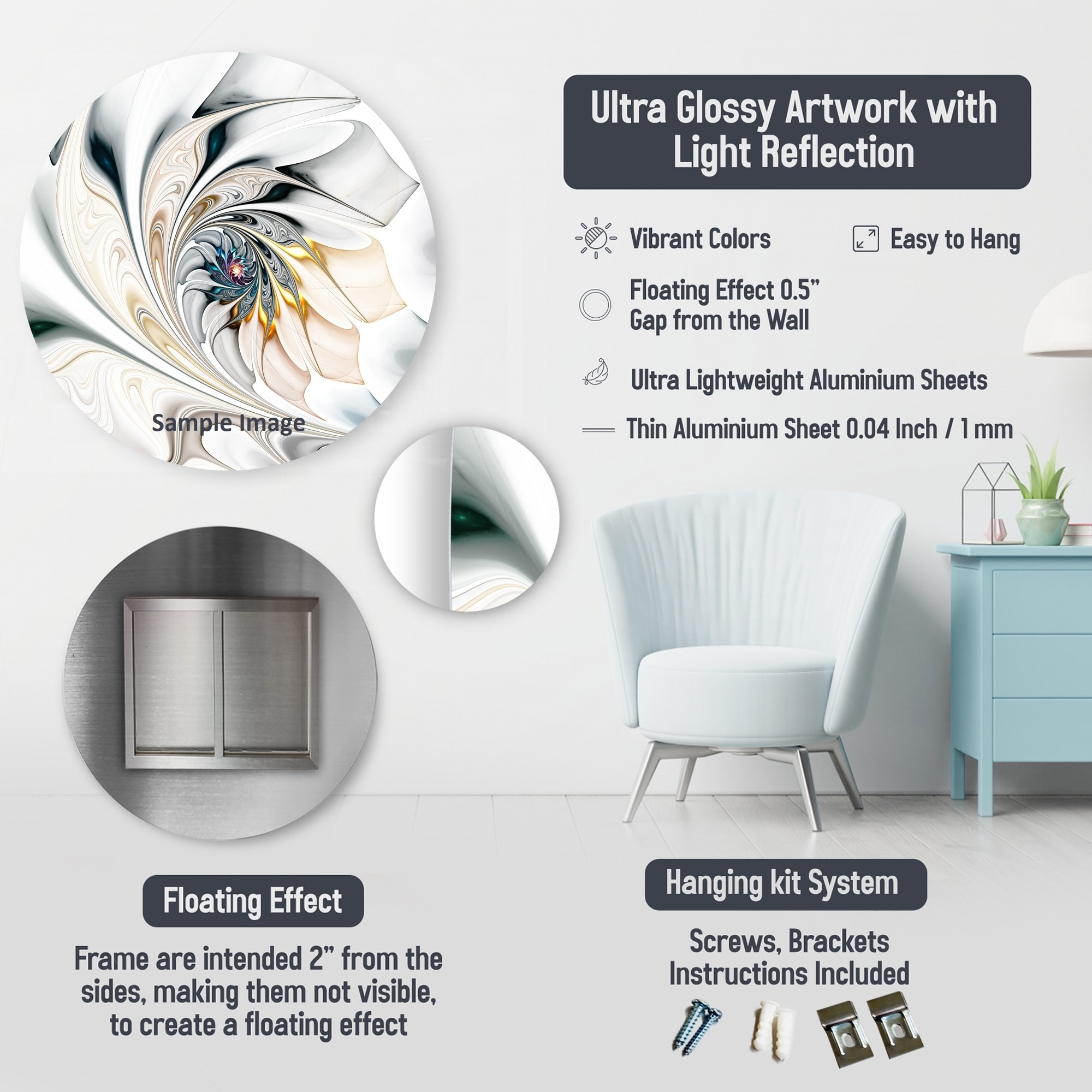The image is a graphic advertisement showcasing an ultra-glossy artwork product with light reflection. Positioned in the top right corner is white text within a gray rectangle that reads "Ultra Glossy Artwork with Light Reflection." Below this, a detailed list of product features is provided, including "Vibrant Colors," "Floating Effect 0.5 inches gap from the wall," "Easy to Hang," and "Ultra Lightweight Aluminum Sheets," with specifications denoted as "Aluminum Sheet 0.04 inch / 1 millimeter." Underneath, additional text notes the inclusion of a "Hanging Kit System." The background features an interior scene with light blue walls, a white chair, and a light blue dresser. On the right side, there are circular cutouts that presumably display images of the artwork, illustrating the product features. The overall layout suggests a premium product, potentially targeting a middle-class market, though it may benefit from a more minimalistic design to reduce clutter.